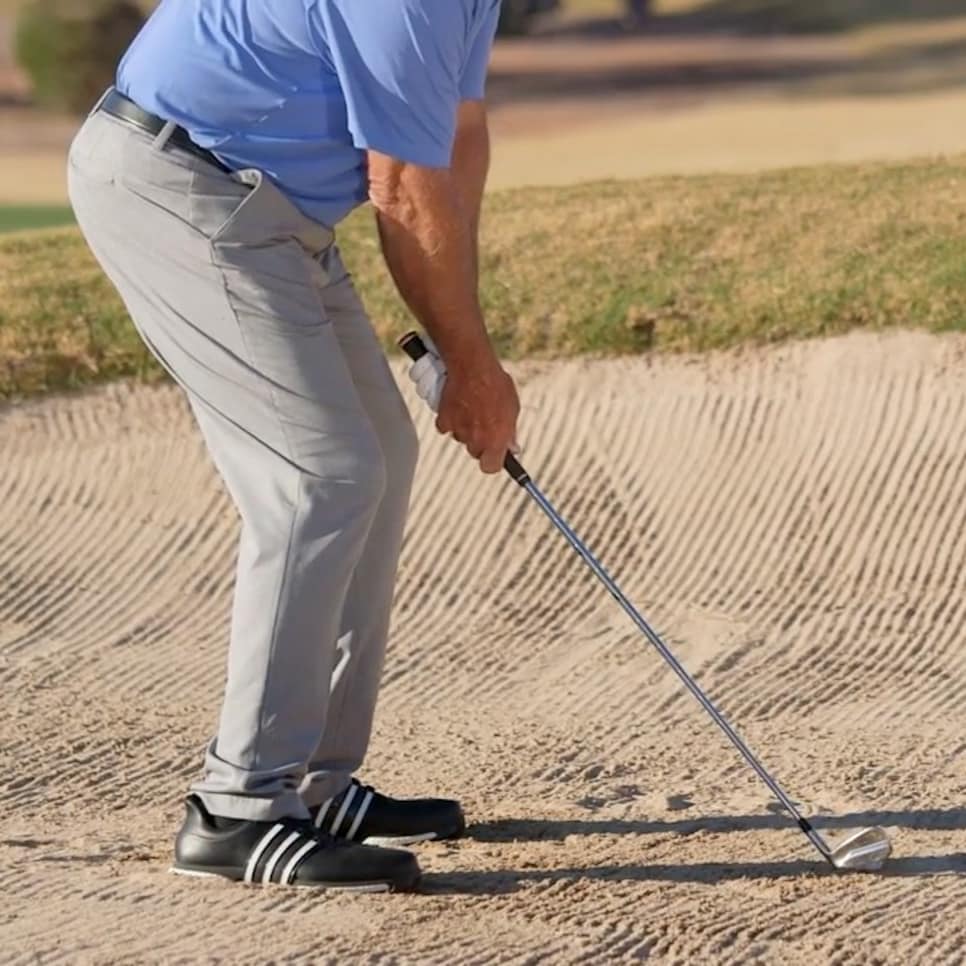In this detailed image, we see a man on a golf course, captured from the waist down as he prepares for a shot. He is wearing a blue shirt and gray khaki pants, secured with a black belt. His footwear consists of black Adidas golf shoes adorned with white stripes. The man grips a metal golf club with a black handle, wearing one golf glove. The sandy terrain of a bunker surrounds him, with patches of brown and green grass visible in the distance, hinting at the expansive golf course beyond. The background appears slightly blurred, focusing attention on the golfer's poised stance and equipment.